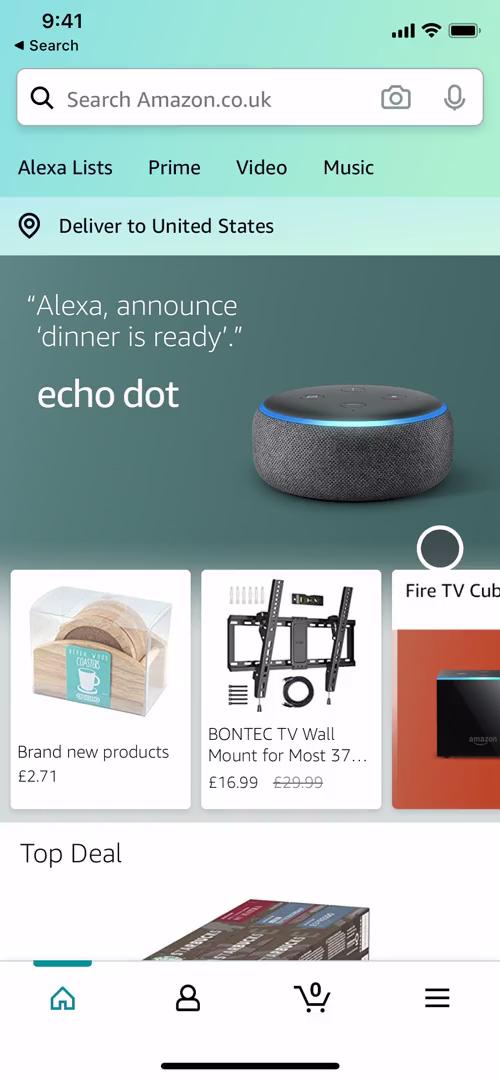This image is a detailed screenshot of the Amazon mobile interface on either the Amazon mobile website or app, viewed from a mobile device.

**Top Section:**
- **Status Bar:** Displays the time (9:41 AM) in black on the left. On the right, it shows a full signal bar, full Wi-Fi connection, and a completely charged battery icon, all presented on a gradient background transitioning from light blue to an even lighter blue.
- **Navigation Bar:** Directly below the status bar, on the left, there's a "text search" label with a left-pointing triangle arrow beside it. Following this, a search input field occupies the full width, characterized by a rectangle with rounded corners, a thin gray border, and a white background. Inside the search bar, a gray search icon is on the left, followed by the placeholder text "search Amazon.co.uk" in lighter gray. On the right side of the search field are a camera icon and a microphone icon for additional search functionalities.
- **Feature Navigation:** Below the search bar, a navigation panel includes four options: "Alexa," "Lists," "Prime," and "Video" written in title case, with black text-center alignment, on the same blue gradient background.

**Middle Section:**
- **Delivery Information:** A new section begins with a light blue background indicating "Delivered to United States" accompanied by a location icon on the left.
- **Featured Product:** Below the delivery info, an image of the Amazon Echo Dot is set against a slate gray background, with the text "Alexa, announce dinner is ready" in white. A white circle with a dark center, typical of the current tab indicator of the web browser, appears below the Echo Dot image.

**Bottom Section:**
- **Product Categories:** Three product images are displayed side by side:
  - **First Product:** Features an item in a wooden box, labeled "Brand new products" and priced at "271 euros."
  - **Second Product:** Displays a black TV wall mount, described as "Bond Tech TV wall mount for most 37..." and priced at $16.99.
  - **Third Product:** Shows the Fire TV Cube, though partially obscured. 

- **Top Deals:** The beginning of another section is visible, marked "Top deal" on a white background with the top edge of a product peeking through, but the screen ends here.

**Navigation Bar:**
At the very bottom of the screenshot is the app's navigation bar, featuring icons for Home, User Account, Shopping Cart, and a Menu represented by three horizontal lines.

This captures the interface's structure, media elements, and navigation features comprehensively.